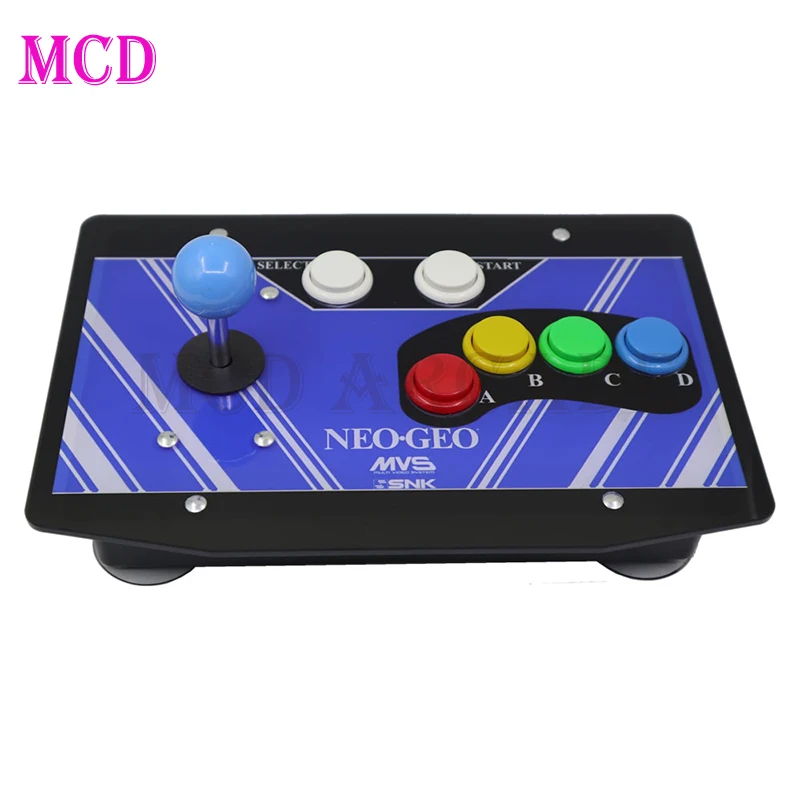This detailed photograph showcases a retro video game controller with a nostalgic design, set against a plain white background. In the upper left-hand corner, a pink text that reads "MCD" stands out. The controller itself features a black outer frame with two rounded feet at the front corners. The top surface has a metallic panel with purple and white chevron patterns, held together by visible screws, adding to its vintage appeal. On the left side of the controller, there is a blue joystick that can be moved in various directions. At the top center, there are two white buttons labeled "Select" and "Start." On the right side, the controller has four colorful buttons: a red button labeled "A," a yellow button labeled "B," a green button labeled "C," and a blue button labeled "D." At the bottom of the controller, metallic lettering reads "Neo Geo MVS SNK," highlighting its classic gaming legacy.